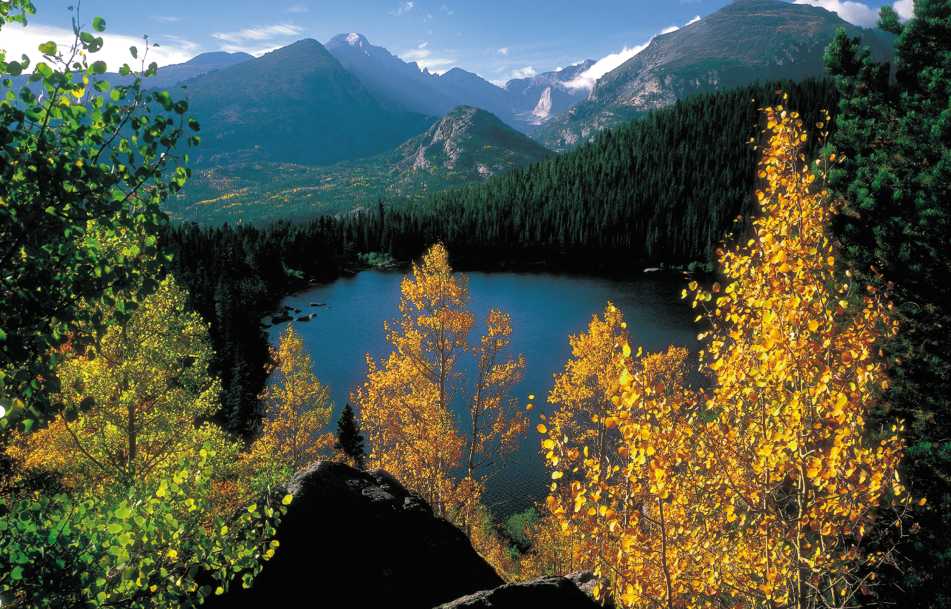This breathtaking aerial photograph captures a stunning panoramic view of a serene lake nestled within mountainous terrain. Taken from a rocky ledge, the foreground features vibrant yellow treetops, signaling the fall season. The circular lake, surrounded by a mix of lush fir trees and a variety of foliage, sits centrally in the image. To the right, the landscape ascends into a hillside cloaked in dense, green pine forest typical of northern environments. Encompassing the lake, distant low-lying hills give way to majestic mountains that stretch across the horizon. A prominent small mountain, encircled by open fields, juts out dramatically in the middle distance. Further beyond, the rugged, jagged peaks of towering mountains rise sharply, with some capped in snow and interwoven with lingering fog. Overhead, a clear blue sky is dotted with scattered clouds, adding to the serene and picturesque nature of the scene.